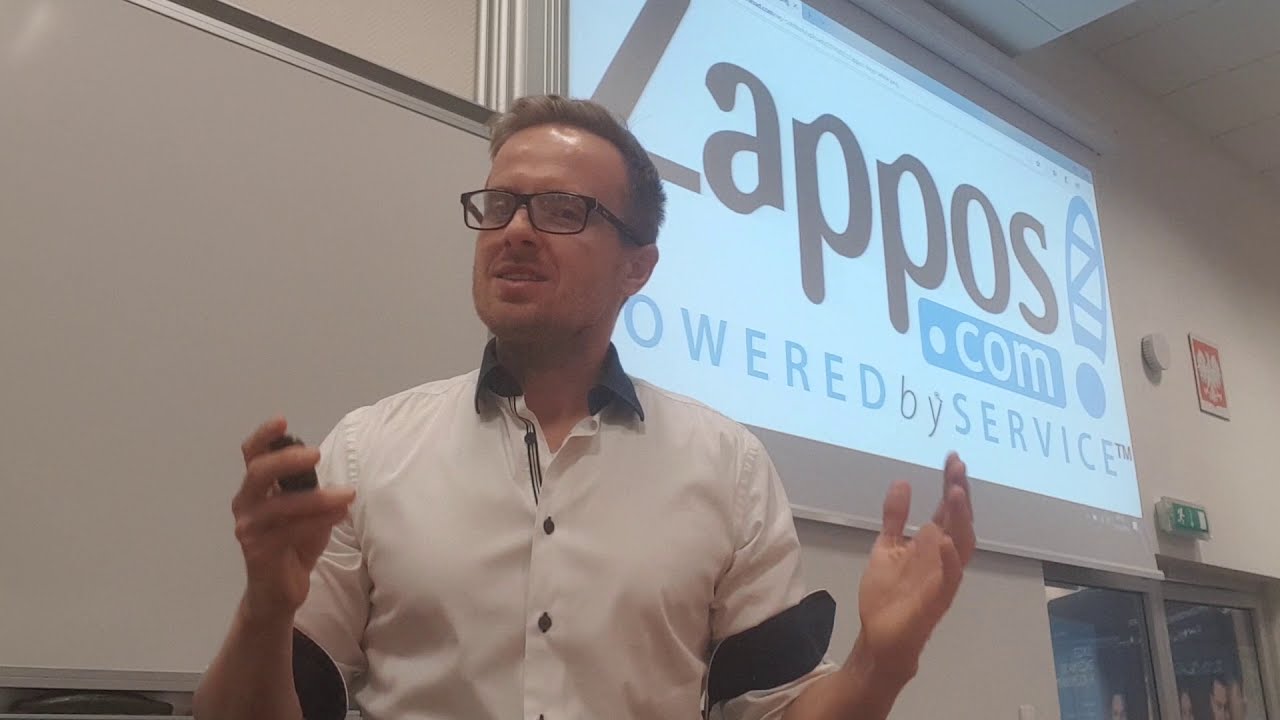A man with a light complexion and slightly curly, light brown hair stands in what appears to be a business setting, presenting in front of a projector screen displaying a PowerPoint slide. The slide prominently features the brand "Zappos.com" with the tagline "Powered by Service" beneath it. The word "Buy" on the slide is highlighted in black while the rest of the text is in blue. The man, whose forehead catches a bit of light making it appear shiny, wears distinctive black-rimmed glasses and a white button-up shirt with black collars and sleeves. His right hand, holding a black remote, is at shoulder height in an explanatory gesture, while his left hand is open and slightly extended. The background includes a white wall, a whiteboard to his left, and sliding glass doors with a green sign above them along with an air filtration unit and a fire alarm to his right. The overall setting is well-lit, providing ample natural light, suggesting it is daytime.